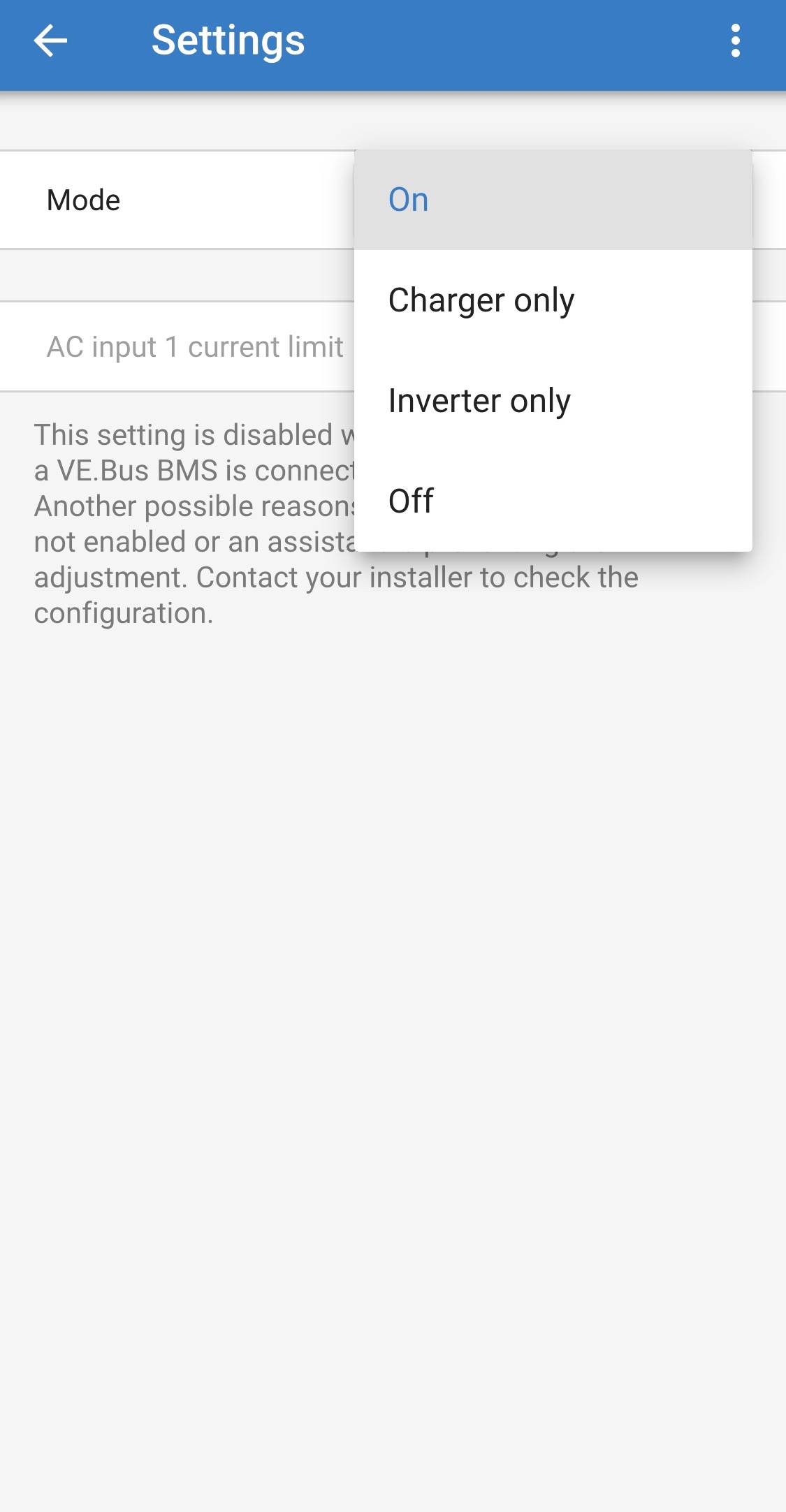The image displays a phone or tablet screen featuring a hierarchical user interface layout. At the top, there is a blue bar with a white left-pointing arrow followed by the word "Settings" in white text. On the far right of the bar, three white dots are vertically aligned. Directly below this bar is a narrow light grey strip, which is then followed by a white strip labeled "Mode" on the left in black text. Another light grey strip appears beneath this, followed by a white strip that reads "AC Input 1 Current Limit" in grey text.

The remaining portion of the screen is light grey, with various informational texts. A small pop-up square is present, partially obscuring the background text. Visible behind this pop-up, the text includes messages such as "This setting is disabled," "VE.BUS BMS is connect," and "Another possible reason, not enabled or an assist, adjust." It also suggests contacting "your installer to check the configuration."

In the pop-up square itself, the word "On" appears at the top in blue and is highlighted in grey. Below this header, the white section of the box presents three options in black text: "Charger Only," "Inverter Only," and "Off."

Overall, this detailed and structured layout provides a clear navigation scheme and options for the user, potentially regarding power management settings.